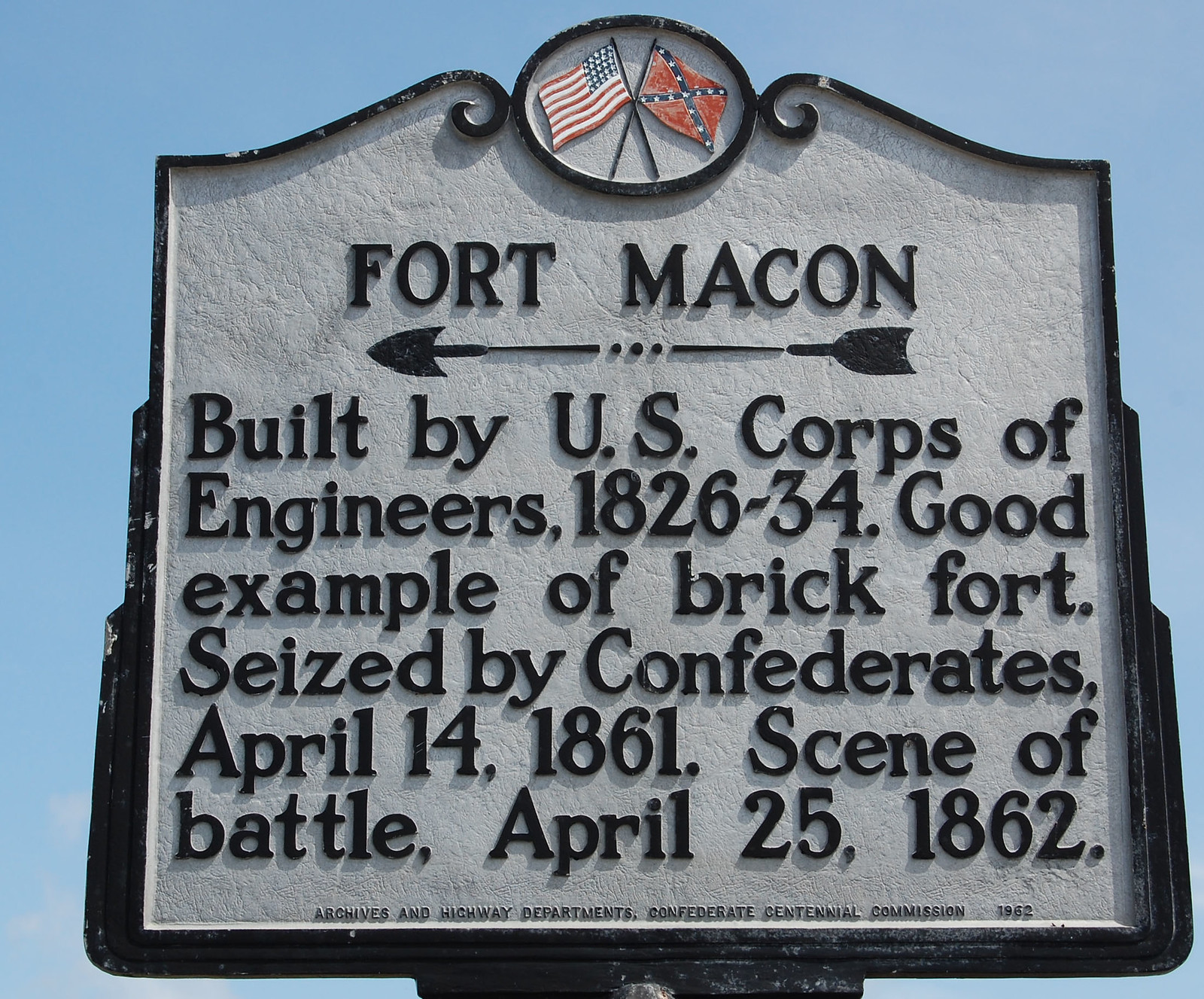The image shows a monument or plaque of a dark gray color with a black outline around its border. At the very top, it features a circle with an American flag tilted to the left and a Confederate Dixie flag, also tilted, to the right. The sign is for Fort Macon, spelled M-A-C-O-N, with a black arrow pointing to the left, resembling an arrow from a bow. 

Below the title, the text continues in black writing: "Built by U.S. Corps of Engineers 1826 to 34. Good example of Brick Fort. Seized by Confederates April 14, 1861. Scene of battle April 25, 1862." 

At the very bottom, in much smaller and hard-to-read text, it says: "Archives and Highway Departments Confederate Centennial Commission, 1952," though the last part might be 1962 due to the small font size. The entire monument is stylistically bordered and set against a clear blue sky. The sign’s core, the non-words area, appears to be made of rough gray stone.